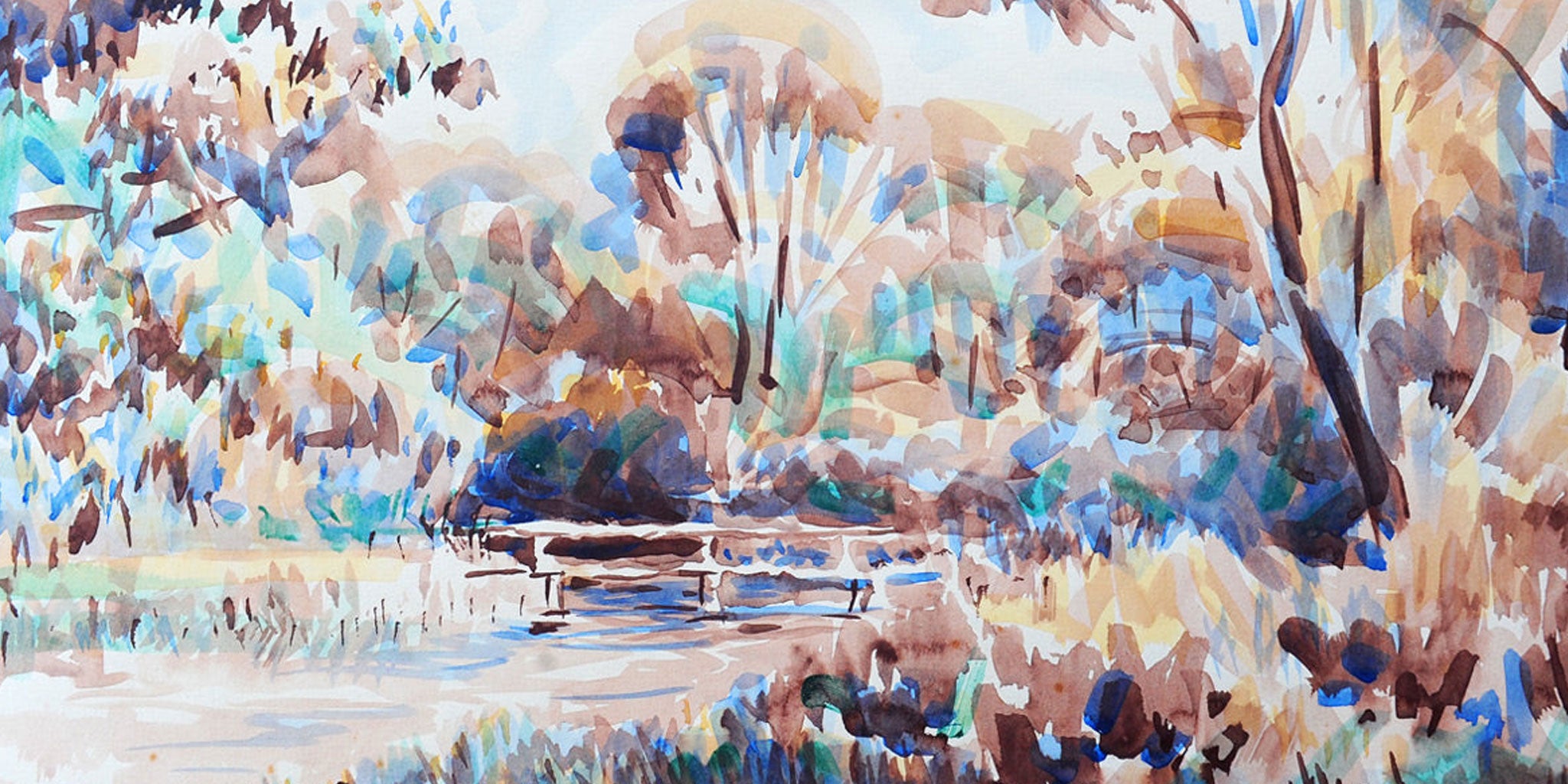This captivating watercolor and digital artwork, rendered in an abstract and impressionistic style, portrays an outdoor scene featuring a small wooden footbridge spanning a creek or river. Dominated by hues of brown, beige, and orange with accents of blue and green, the scene conveys a sense of a wetland or marshland environment. The painting's unique palette choice contrasts with typical expectations, using orange and brown as primary colors while blue and green play supporting roles. The creek meanders from the bottom left towards the center, overlaid by the bridge with its white and brown highlights. Surrounding the waterway, the lush scenery consists of trees, tall grasses, and possibly flowers, depicted with bold, individual brushstrokes that emphasize the textured foliage. In the background, more trees and bushes can be seen, with something hanging from a tree that could be interpreted as a treehouse or birdhouse. The sky peeks through in white and light blue, enhancing the overall ethereal and imaginative quality of the landscape.